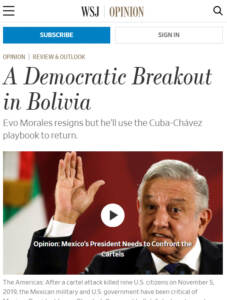Homepage for an Opinion Piece:

The homepage features a clean, white background with a minimalistic design. In the upper left corner, three horizontally stacked lines serve as a menu icon. Centrally positioned, black text reads "WSJ/" followed by brown text that states "Opinion." In the far upper right corner, a black magnifying glass icon provides a search function.

A light gray line extends from left to right beneath this header. Below the gray line are two icons placed side by side: a blue rectangle with white text that says "Subscribe," followed by a white rectangle with black text that says "Sign In."

Further down on the left side, brown text reads "Opinion/," which is followed by black text that says "Review and Culture." Directly beneath this section, the black text headline "A Democratic Breakout in Bolivia" is prominently displayed. In smaller text below the headline, it reads, "Evo Morales resigns, but he'll use the Cuba Chavez playbook to return."

Below this description, a video thumbnail features an elderly man with gray hair, wearing a black suit, white shirt, and dark blue tie. He is waving with his right hand raised above his head. The background of the video is red, and a white, green, gold, and red flag is visible in the left corner.